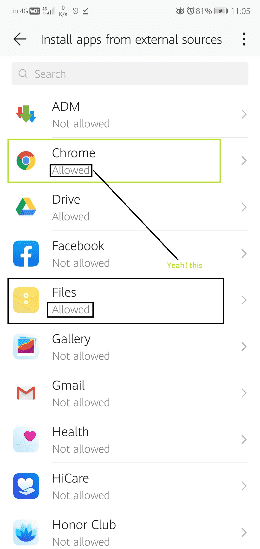The image depicts a smartphone app settings interface. At the top of the screen, various standard icons are visible, showing the signal strength, battery percentage, and current time. There is also a back arrow for navigation. The title reads "Install apps from external sources," indicating the intent of the settings page.

Beneath the title, there is a search function for easy navigation. The interface is organized with a list of apps and their permission statuses. Each app entry consists of the app's name, its icon, and a corresponding permission status highlighted in various colors to draw attention. 

- **ADM:** "Not Allowed," displayed without additional highlighting.
- **Chrome:** "Allowed," with a green-colored box around the app icon and the text.
- A black line with yellow text reads "Yeah this," likely a note or instruction, though its purpose is unclear.
- **Drive:** "Allowed."
- **Facebook:** "Not Allowed."
- **Files:** "Allowed," with black boxes around both the icon and the word "Allowed."
- **Gallery:** "Not Allowed."
- **Gmail:** "Not Allowed."
- **Help:** "Not Allowed."
- **HiCare:** "Not Allowed."
- **Honor Club:** "Not Allowed."

Each app name is followed by a gray arrow, indicating that these entries may be expandable or have additional settings. The majority of the text is black on a white background, ensuring readability. The use of colored boxes and text highlights specific permissions, guiding someone through configuring their smartphone’s app permissions.